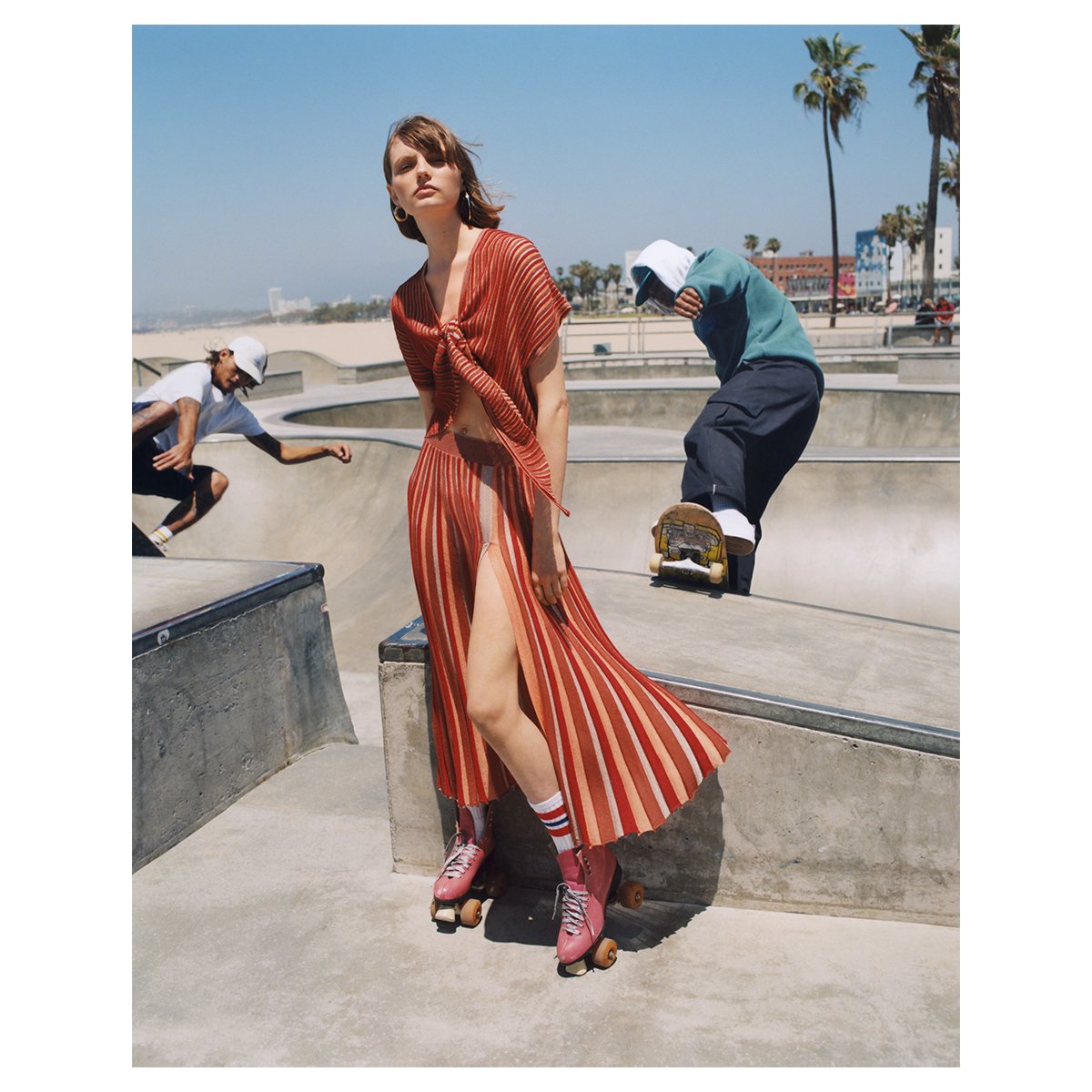In this vibrant and dynamic image set at a skate park in California, a young woman in her early 20s serves as the focal point. She stands confidently in the middle of the frame, modeling a striking 70s-inspired flowy dress adorned with vertical stripes in shades of orange, red, tan, and brown. The dress features a high slit that reveals her leg, adding a touch of allure to her retro ensemble. Complementing her outfit, she dons pink roller skates with white laces and tall white socks accented with red and blue stripes, reminiscent of 80s fashion. Her short, straight brown hair falls just to her shoulders, and she accessorizes with large gold hoop earrings in each ear.

To her left and right, two young male skateboarders are captured mid-action, grinding on a rail atop a ramp. One skateboarder, dressed in a green sweatshirt over a white hoodie and black pants, adds to the energetic atmosphere of the skate park. The backdrop reveals tall palm trees and distant buildings, situating the scene near the iconic Californian coastline. The colors in the image range from blue-green, sky blue, and sandy gray to peach, beige, and various earthy tones, enhancing the overall vividness of the setting.

The concrete park and the lively beachside ambiance lend themselves perfectly to this captivating and dynamic shot, blending fashion, sport, and the laid-back Californian lifestyle.